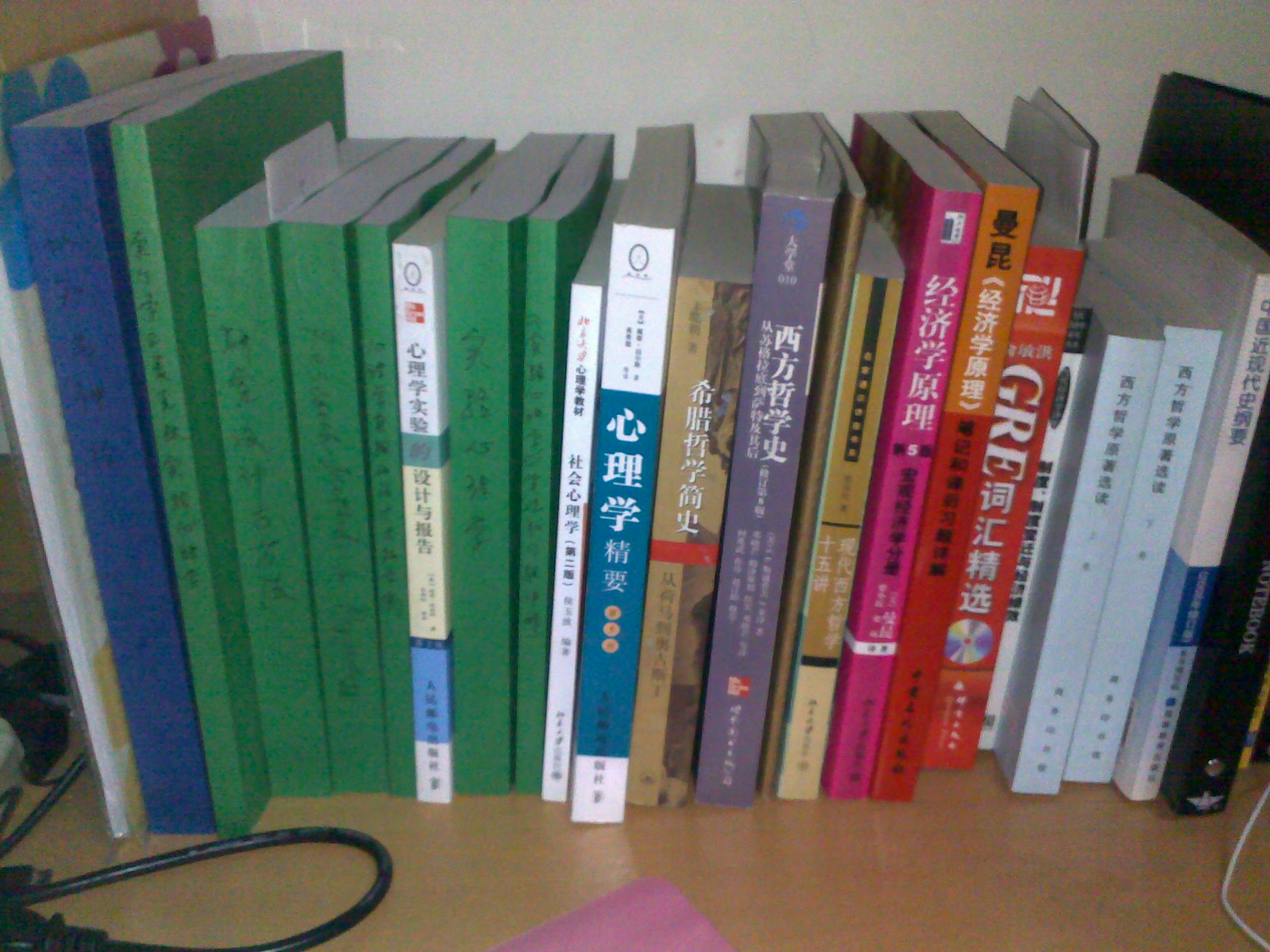This color photograph captures a close-up of a bookshelf filled with an array of predominantly Asian-language books, most likely Chinese or Japanese. The bookshelf, which appears to be made of light brown glossy wood, reveals a well-organized collection with mostly matte covers in solid colors. From left to right, the books vary in color and height, prominently featuring several Kelly green and bright blue books. Interspersed among these are books with more traditional, commercially printed designs, boasting complex graphics and a mix of colors. Notable among them is a red book with the letters "GRE" visible, accompanied by Asian script and a CD symbol.

At the center of the image, a purple post-it note peeks out, while a black cord, likely a computer power cable, arcs into the scene from the left corner, with a bit of a white cord appearing on the right. The scene is framed against a white back wall and the brown side of the bookshelf, enhancing the neat arrangement of the books which span from near the top to near the bottom of the shelf.

Among other visible details, there’s a taller white book with a small flower at the top, a series of green and blue books of various thicknesses, some shorter white spined books, a distinctive brown book with a red stripe across its center, a worn-looking purplish book, and a thin gold one. Towards the end of the row, there is a combination of pink, orange, red, and white bound books, with the final book being taller and transitioning from white to dark blue midway down, then fading to light blue. The overall scene is dimly lit and slightly out of focus, lending a cozy yet cluttered atmosphere to this snapshot of a scholarly collection.